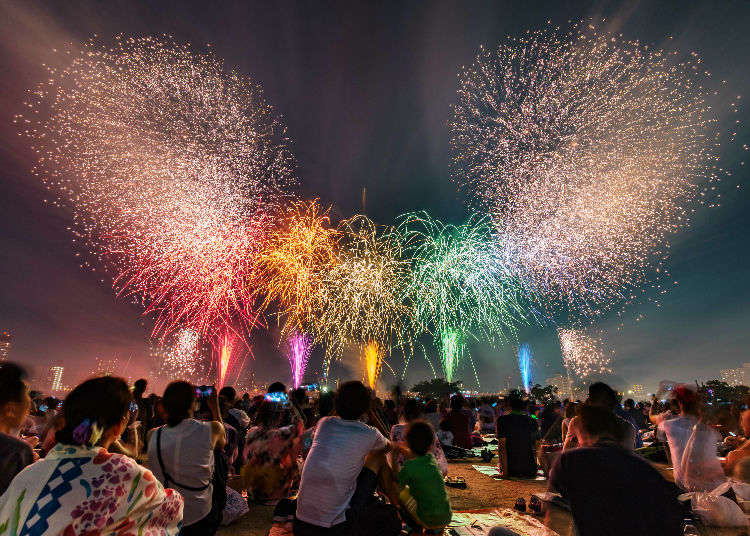This square photograph, potentially captured with a fisheye lens, presents a compelling nighttime scene of a large crowd, approximately 60 to 100 people of varying ages, seated on a grassy field, perhaps in a park. They are watching a vibrant firework display that occupies the top two-thirds of the image. The diverse crowd, some comfortably sitting on picnic blankets and mats, others standing or slightly crouched, watch in awe as multi-colored fireworks light up the sky. Six spectacular sprays of color—orange, red, pink, yellow, green, blue, and gold—illuminate the light gray sky with dazzling patterns. Among the crowd, a woman on the left in a colorful kaftan, her hair adorned with a multi-colored barrette or scrunchie stands out, capturing the magic on her phone. Similarly, numerous spectators have their phones out, documenting the festive atmosphere of this possible holiday or celebratory event.